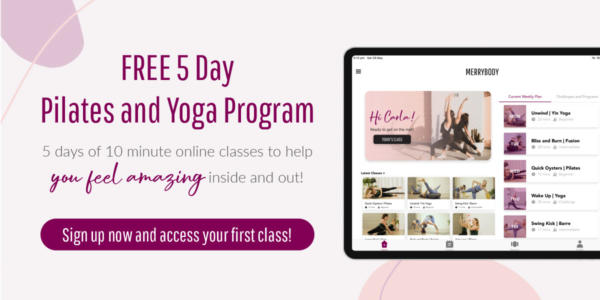Here is a polished and detailed caption for the described image:

---

The advertisement banner for a yoga program features a predominantly white background with playful pink accents, including pink circles and a pink ring. On the left side, the text in pink reads "Free 5-Day Pilots in Yoga Program." Beneath this, additional text details: "5 days of 10-minute online classes to help you feel amazing inside and out." A purple rectangular box with white text invites viewers to "Sign up now and access your first class."

On the right side of the banner, a computer screen is pictured, displaying the program's interface. Though the text on the screen is small, it shows a menu of video classes available for selection. The program is titled "Merry Body," and appears to be personalized, possibly welcoming a user with a high-collar image. The screen depicts a woman performing a yoga pose, with six video thumbnails of various yoga practices lined up beneath her image. The right sidebar also features thumbnails with different yoga poses, indicating that users can browse and select the specific classes they wish to join.